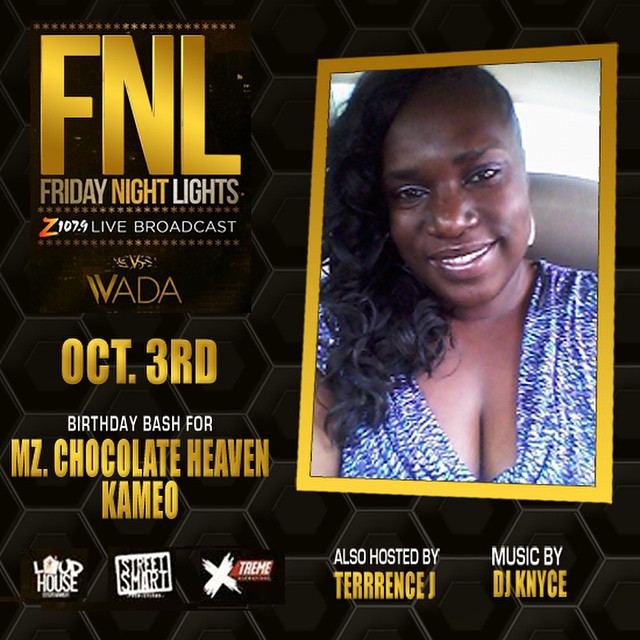The image is an advertisement poster for "Friday Night Lights." On the left side, in large gold letters, it says "FNL," followed by smaller text that reads, "Friday Night Lights," "Z107.9 Live Broadcast," "WADA," "October 3rd," "Birthday Bash 4," and "MZ Chocolate Heaven Cameo." Each line alternates between gold and white text. On the right side of the poster is a picture of an African American woman with long black hair swept to the side, wearing a v-neck, purple shirt speckled with white. She is looking directly into the camera and captured from head to chest. Below the main content, several sponsors' logos are displayed in a line: Loud House, Street Smart, Extreme, “Also hosted by Terrence J,” and "Music by DJ Nice." The entire poster has a black background with a hexagonal pattern.